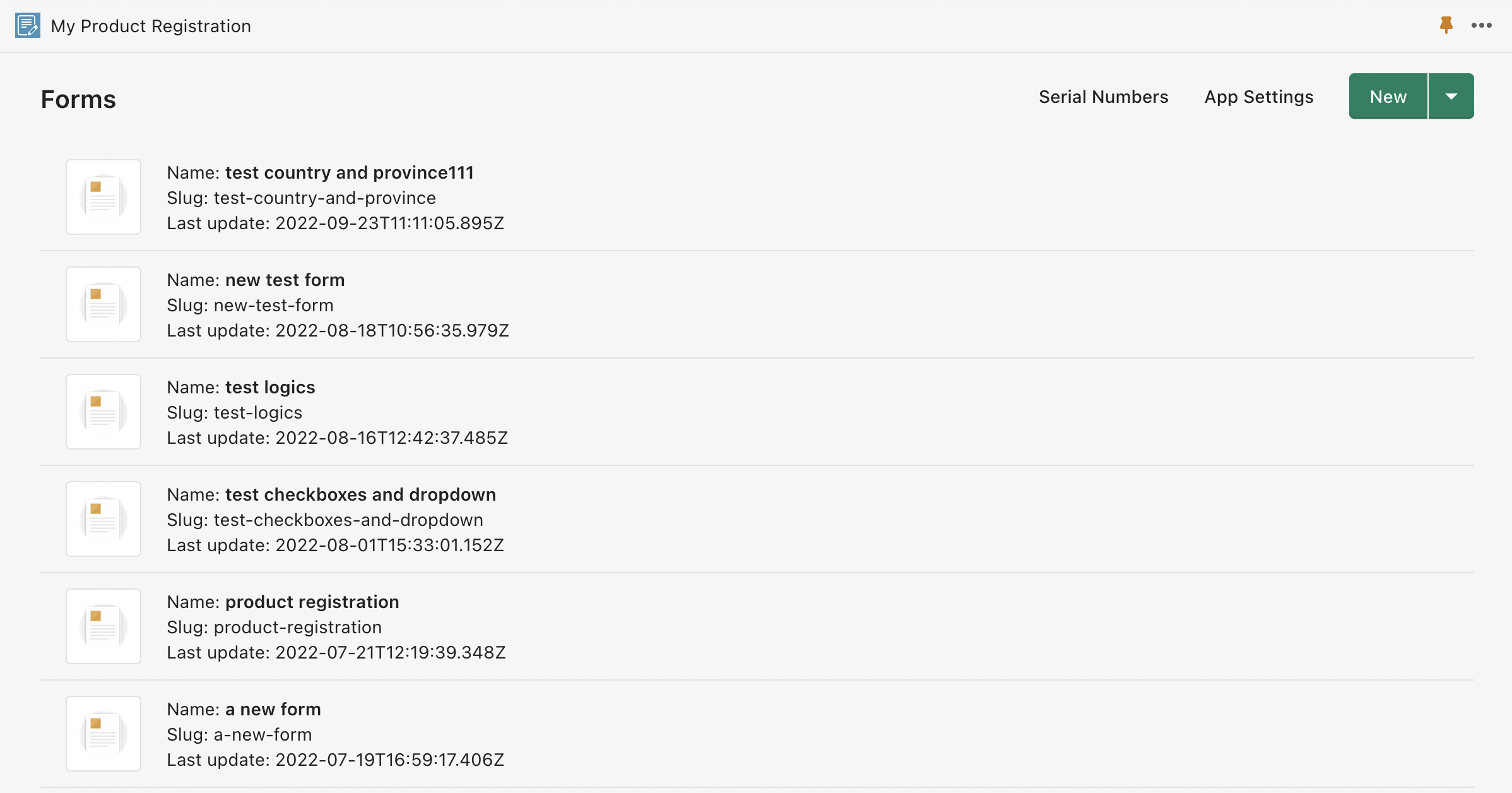This desktop screenshot is predominantly white and lacks any visible browser or OS interface. In the top left corner, there is a blue icon featuring a white-outlined sheet of paper with a pencil, labeled "My Product Registration." To its right is a yellow pushpin and a trio of horizontal dots, likely representing additional settings. The text "Forms" appears nearby, followed by "Serial Numbers," then "App Settings," and a green rectangular box marked "New," accompanied by a drop-down arrow.

The main content area lists various forms, each represented by a white sheet with an orange square in the top left corner. Below is a detailed breakdown of each form:

1. **Form: Name, Test Country and Province 111**
   - **Slug:** test-country-and-province
   - **Last Update:** 23rd September 2022 at 11:11:05.895Z

2. **Form: New Test Form**
   - **Slug:** new-test-form
   - **Last Update:** 18th August 2022 at 10:56:35.979Z

3. **Form: Test Logics**
   - **Slug:** test-logics
   - **Last Update:** 16th August 2022 at 12:42:37.485Z

4. **Form: Text Checkboxes and Drop-Down**
   - **Slug:** text-checkboxes-and-drop-down
   - **Last Update:** 1st August 2022 at 15:33:01.152Z

5. **Form: Product Registration**
   - **Slug:** product-registration
   - **Last Update:** 2nd July 2022 at 12:19:39.034Z

6. **Form: A New Form**
   - **Slug:** a-new-form
   - **Last Update:** 19th July 2022 at 16:59:17.4067Z

Although labeled "Product Registration," it appears to be a collection of varied forms rather than actual product registrations.